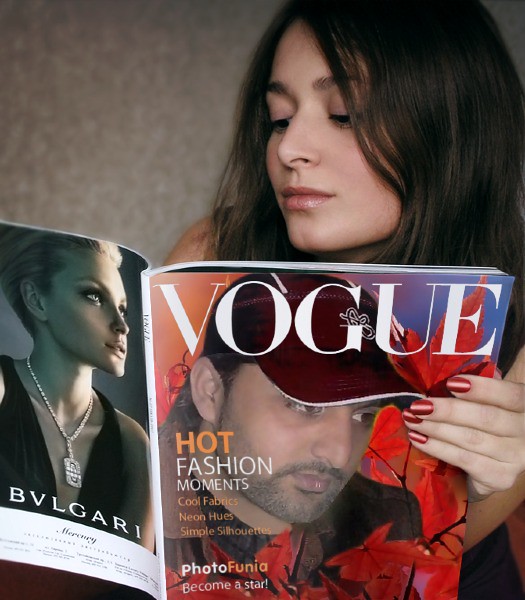A young woman with predominantly fair skin and slightly wavy, dark brown hair is engrossed in reading a Vogue magazine. The wall behind her is a muted blend of gray and brown tones. She holds the magazine with her left hand, showcasing her shiny, red-painted nails. Her face and one of her hands are partially visible as she looks down at the magazine. The magazine's cover features a Middle Eastern man with dark skin, a dark beard, and a burgundy hat with white trim, surrounded by autumn leaves. The cover of the magazine also includes white text that reads, "Hot Fashion Moments." On the back page, there is an advertisement for Bulgari, depicting a blonde woman with short hair, wearing a black gown with straps, and showcasing a luxurious silver and diamond necklace.